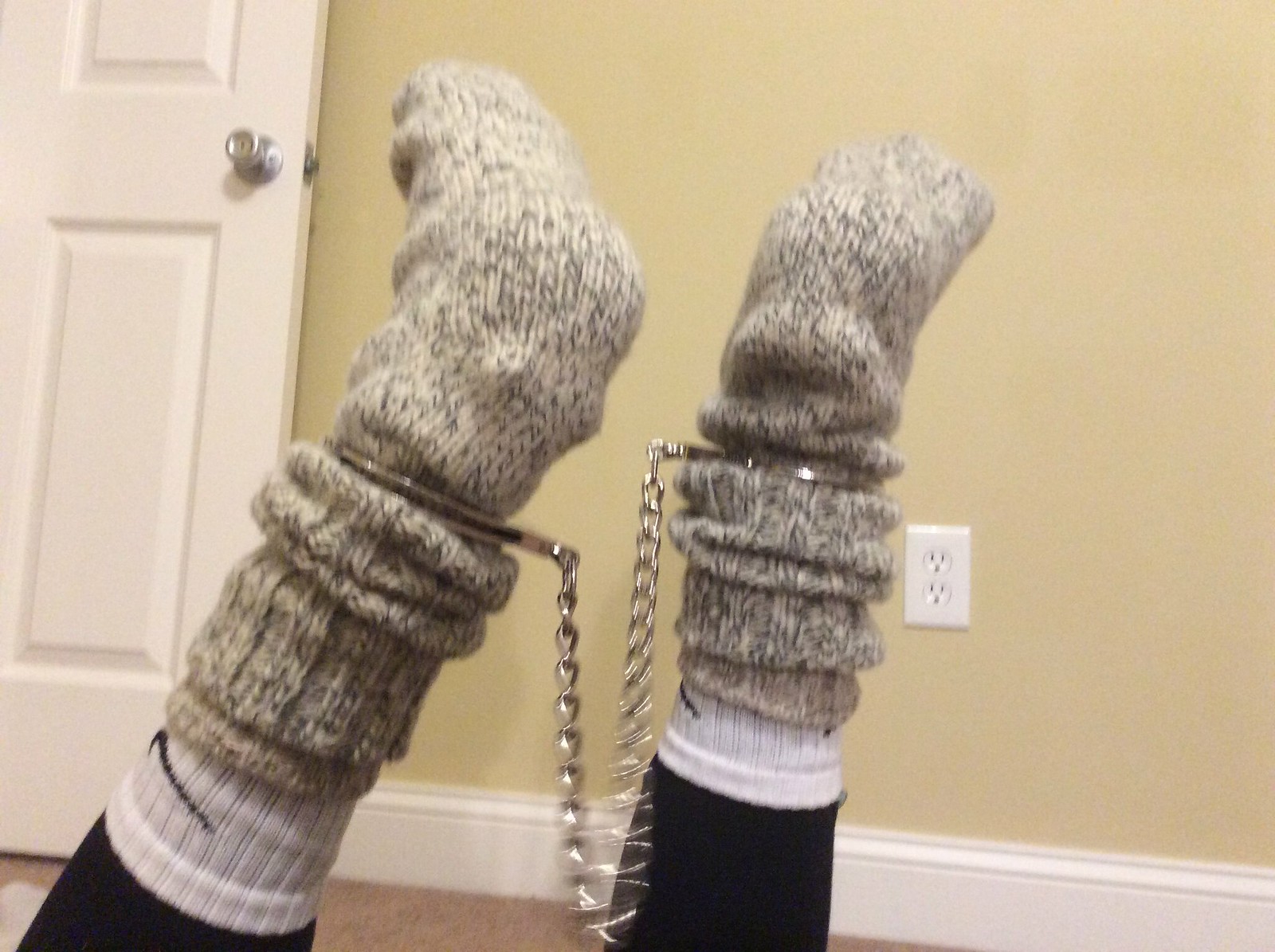This photograph features a pair of feet and calves sticking straight up from the bottom, nearly reaching the top of the image. The legs are clad in black leggings or spandex, and the feet are covered in white socks, each displaying a Nike logo. Over these, the person wears heavy, variegated brown and gray wool socks. Silver handcuffs with a chain between them are tightly fastened around the ankles. The background reveals a cream or light tan wall with a white baseboard and a white electrical outlet centrally positioned near the lower part of the wall. To the left, there is a partially open white door featuring a silver doorknob. The floor is dark brown, and there is some mention of brownish carpet. The chain in the handcuffs appears slightly blurry, adding to the intricate details captured in this scene.